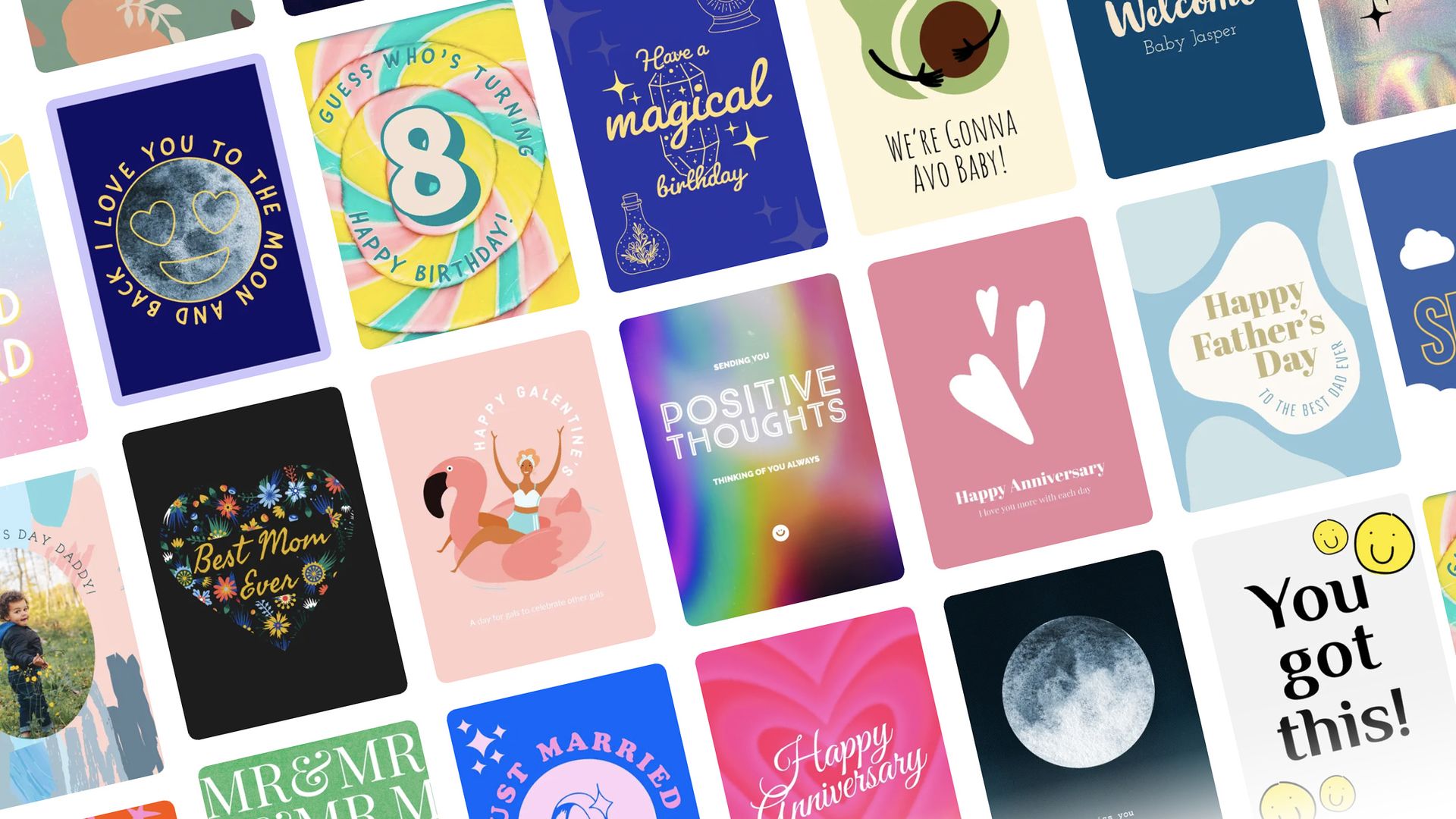In this image, a large white sheet serves as a backdrop for an array of colorful greeting cards, each adorned with unique designs and messages. One card reads "Love you to the moon and back," featuring a cheerful smiley face on a crescent moon. Another celebratory card exclaims, "Guess who's turning eight, Happy Birthday," embellished with whimsical yellow, pink, and blue swirls.

A purple card wishes a "Have a magical birthday," while a playful "We're gonna avo baby" card showcases a cute avocado illustration. The welcoming "Welcome baby Jasper" card stands out in serene blue hues.

For Father's Day, a blue card with white spots sends heartfelt wishes, while a purple card with white hearts marks a "Happy Anniversary." A vibrantly decorated card, filled with swirling colors—purple, blue, green, yellow, red, and pink—promotes "Positive thoughts."

A leisurely-themed card depicts a person lounging on a pink float in a pool, and another blue card proudly hails "Best Mom Ever" with a matching blue heart. Yet another "Happy Anniversary" card appears in a soft pink.

A striking blue card features a prominent, glowing moon, conveying a sense of wonder. Adding to the mix, a white card scattered with bright yellow smiley faces offers encouragement with the phrase "You got this." Each card is uniquely adorable, contributing to a vibrant and joyful collection.